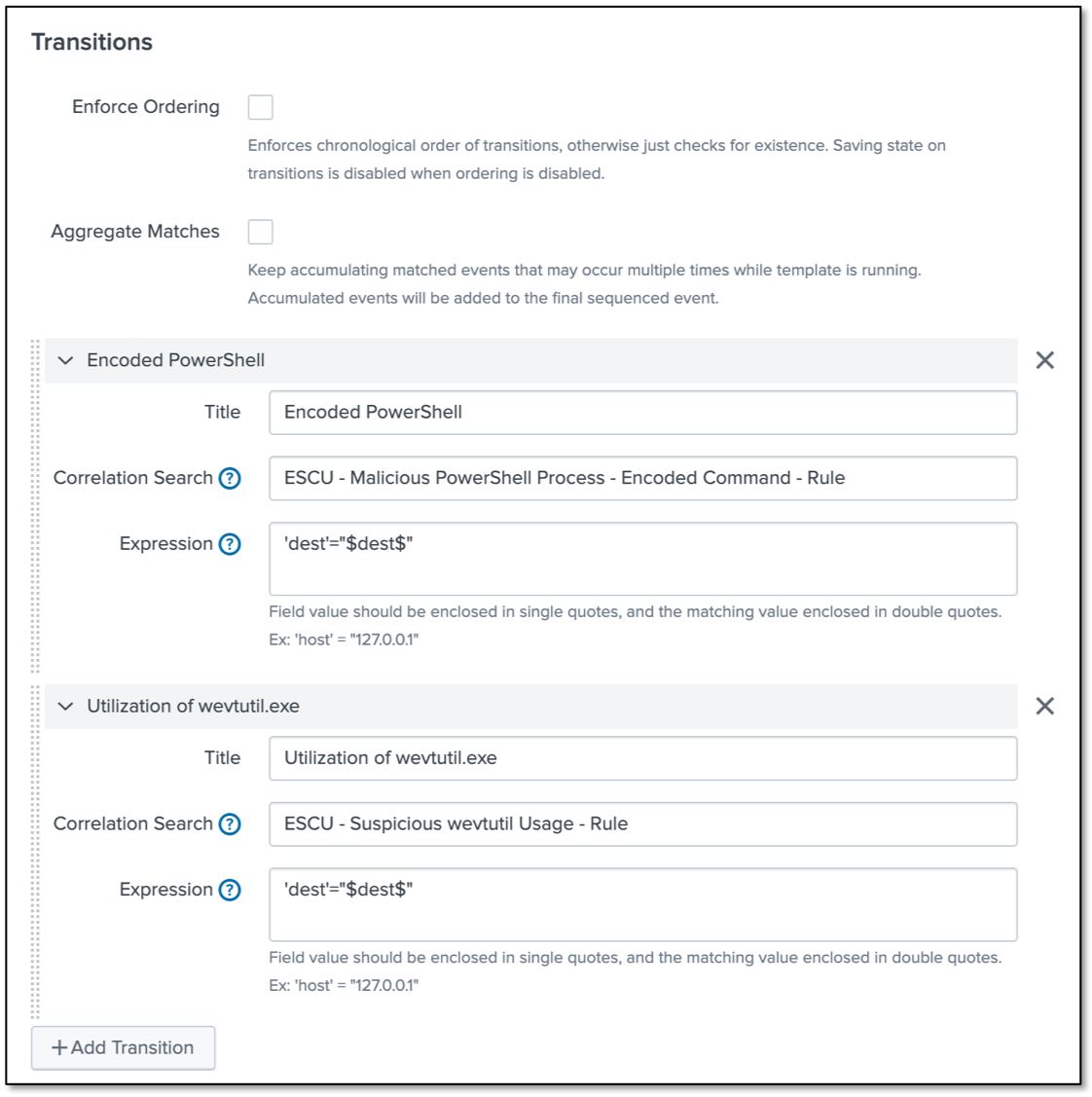The page features a white background with a structured layout. In the upper left corner, "Transitions" is prominently displayed in bold black text. Directly below this header, in slightly smaller black text, is the option "Enforce Ordering" accompanied by a square checkbox. An explanatory note follows: "Enforces Chronological Order of Transitions. Otherwise, just checks for its existence. Saving State on Transitions is disabled when Ordering is disabled."

Below this section, aligned to the left, is "Aggregate Matches," which is also paired with a checkbox. There is a subsequent detailed description: "Keep accumulating matched events that may occur multiple times while a template is running. Accumulated events will be added to the final sequenced event."

The page is visually divided by light gray rectangles that span from left to right. The first rectangle begins with a downward directional arrow on the left, followed by the header "Encoded PowerShell" in bold black text. Beneath this, there is a smaller header titled "Title: Encoded PowerShell," followed by another section labeled "Correlation Search" with a question mark inside a circle for additional information. Next is "ESCU: Malicious PowerShell Process Encoded Command Rule.”

This section is succeeded by a subgroup titled "Expression" (again with an info question mark), followed by the placeholder "DEST = $DEST $". The following instruction notes that "field values should be enclosed in single quotes, and the matching value enclosed in double quotes. Example: host '127.0.0.1'."

A second light gray rectangle follows, also extending from left to right. It too starts with a downward directional arrow on the left and features the text "Utilization of Web2TIL.exe." Beneath this header is a sub-heading "Title: Utilization of Web2TIL.exe," followed by a section labeled "Correlation Search" (with the info question mark). This part is titled "ESCU: Suspicious Web2TIL Usage Rule.”

The pattern continues with the "Expression" section (including the info question mark) and reiterates the placeholder "DEST = $DEST $". Below this, the guiding instruction for field values appears again: "field values should be enclosed in single quotes, and the matching value enclosed in double quotes. Example: host '127.0.0.1'."

In the bottom left corner of the page, there is a rectangular button labeled "Add Transition," completing the cleanly structured layout.